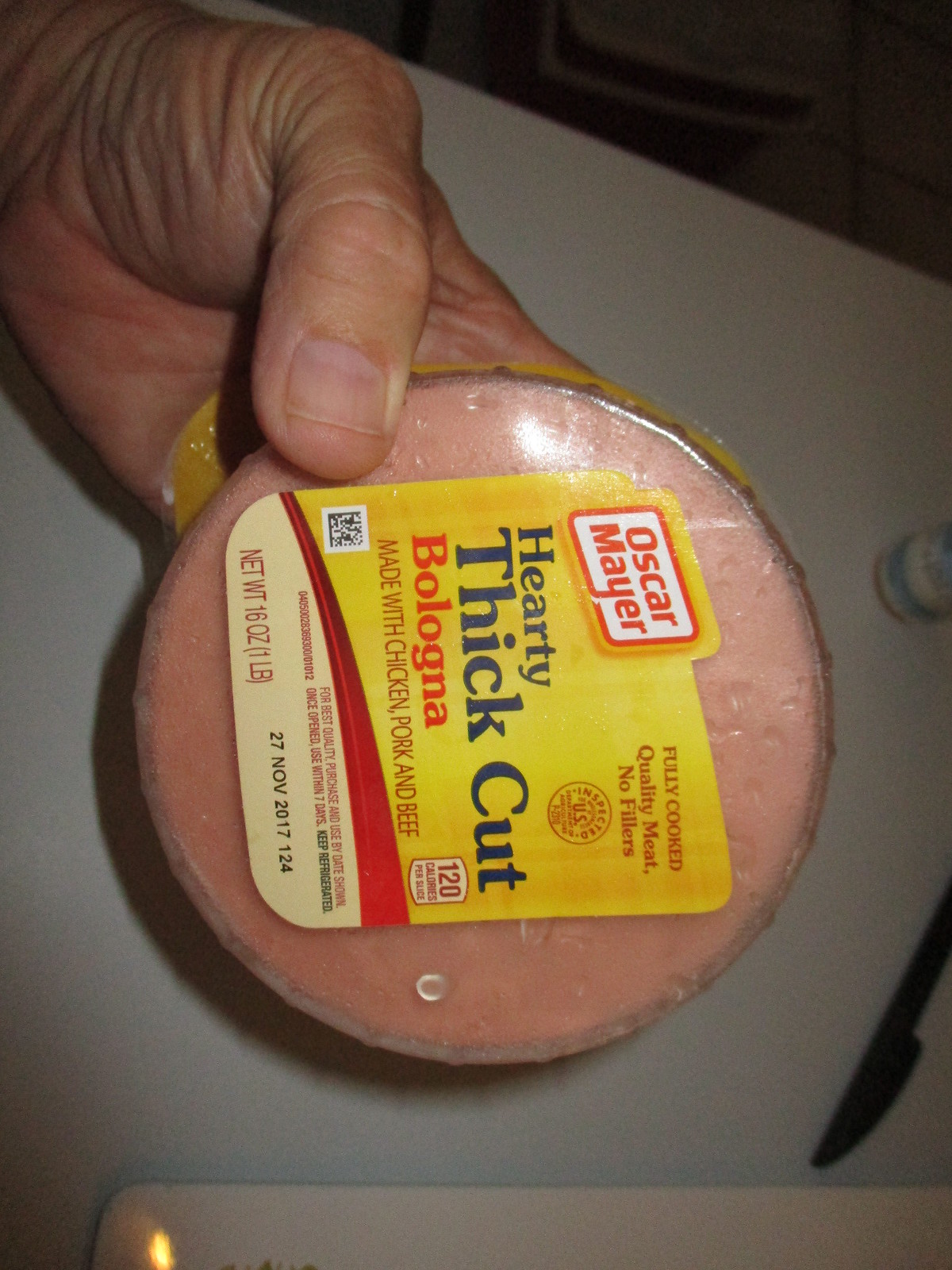In this detailed image, we see a decent-quality, slightly dated photograph of a hand holding a package of Oscar Mayer hearty, thick-cut bologna. The bologna, round in shape, is the focal point of the image and remains in its bright yellow-labeled package. The label, though tilted with the text oriented towards the left, clearly reads "Oscar Mayer" in red, followed by "hearty, thick-cut bologna made with chicken, pork, and beef". The label also states "fully cooked, quality meat, no fillers" and specifies "120 calories per slice" alongside the net weight of 16 ounces and a date of "27 November 2017". The background features a white table, a black plastic knife, a small bottle that resembles a tiny paint bottle, and what appears to be a plate, providing a domestic kitchen setting for the scene.